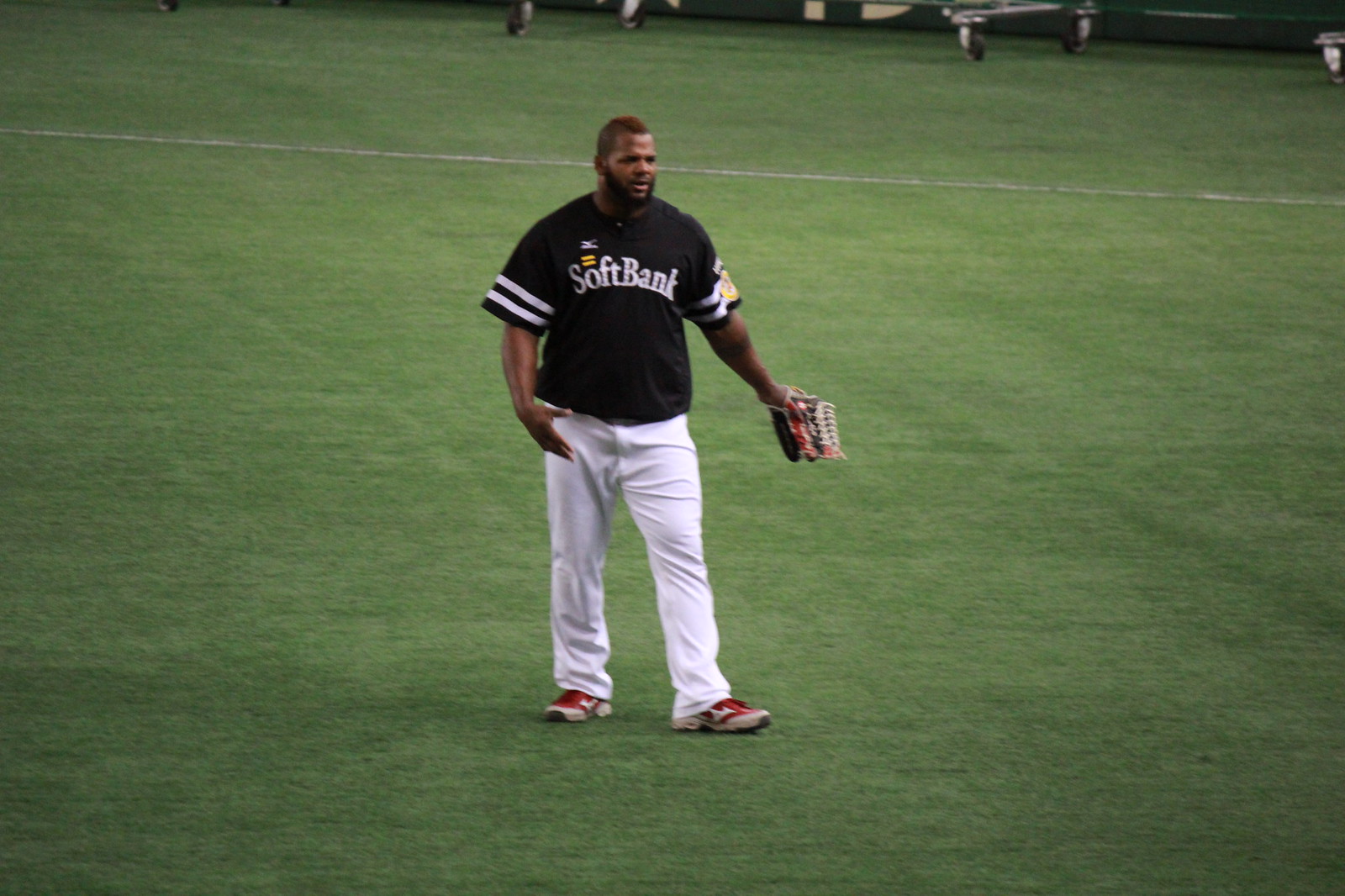In the photograph, an African-American man with short black hair and a slight black beard stands prominently on a green baseball field. He is wearing a short-sleeved black shirt with two horizontal white stripes on each sleeve and the word "SoftBank" emblazoned across the chest in white letters. Complementing his shirt, he wears white uniform pants and red Nike tennis shoes with white tips and soles. His stance, slightly angled to the right, shows his right hand at his side while his left hand extends outward, holding a catcher's mitt that is red and black with white lacing. He appears to be in anticipation, possibly preparing to throw out the first pitch. In the background, a white foul line can be seen stretching from the upper left of the image towards the right. At the top of the image, wheels and metal equipment, possibly carts, are visible next to what seems to be the seating area.